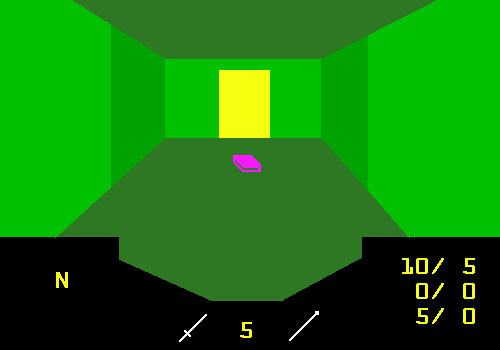In this rectangular image, we are presented with a digital depiction of a room, potentially originating from a video game. The room features a dark green, rectangular floor, surrounded by three bright green walls on the left, right, and rear sides. Centered on the back wall is a yellow, rectangular door. Positioned on the floor directly in front of this door is a small purple book. 

Overlaying the bottom of the image is a score display on a black background. On the right side, yellow text reads from top to bottom: "10," "5," "0/0," and "5/0." At the center bottom, the number "5" is prominently displayed. On the lower left of the image, the letter "N" appears in yellow.